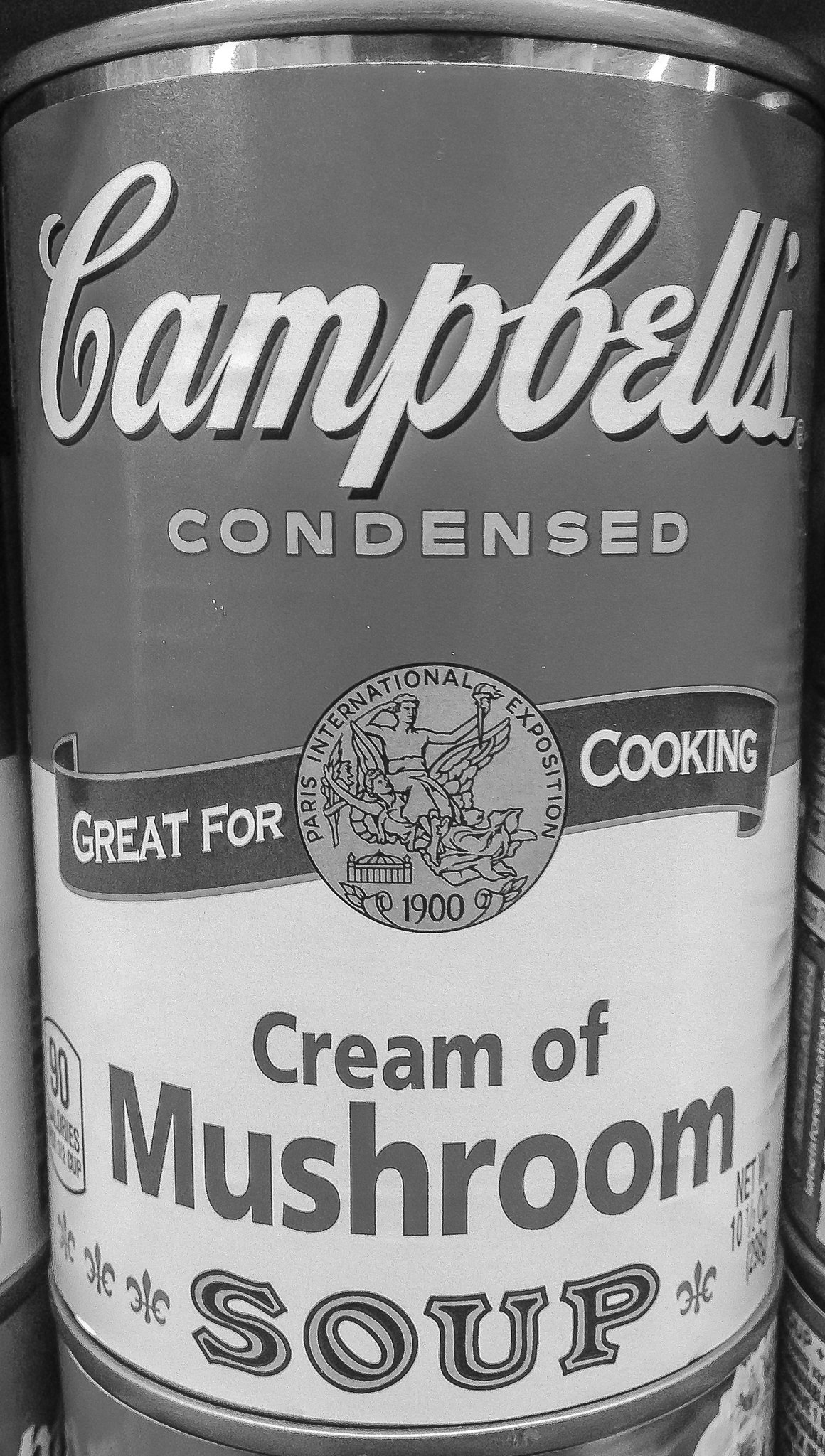A detailed, cleaned-up version of the descriptive caption could be:

"This black-and-white photograph features a can of Campbell's Cream of Mushroom Soup. The can is made of metal, identified by the fine line around the rim, and is wrapped in a paper label. The top of the label prominently displays the word 'Campbell's' in cursive script. Directly below, the word 'condensed' is printed in plain text. A smaller label beneath 'condensed' reads 'great for cooking' in white text. 

At the center of the label, there is an intricate circular emblem referencing the Paris International Exposition of 1900. Inside this emblem, a man ascends alongside cherubs. Directly beneath this emblem, the words 'cream of mushroom' appear, followed by 'soup.' The label also specifies the net weight of the can as 10 ounces, and is adorned with a fleur-de-lis on either side of the word 'soup,' adding to the decorative detail of the label."